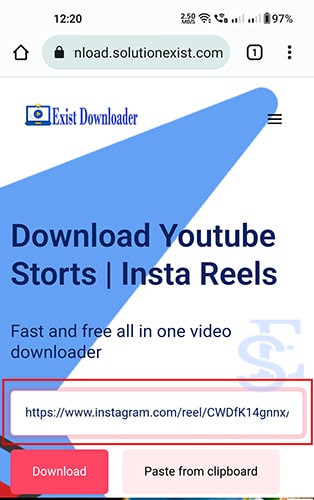The image depicts a promotional website for a browser extension designed to assist users with downloading videos from YouTube and other platforms. The background is white with a blue spotlight effect radiating from the upper right corner to the lower left. At the top of the page, the product name "Exist Downloader" is displayed in bold blue lettering, accompanied by a small icon.

Prominently featured across the blue spotlight area and extending to the right margin is the text "Download YouTube." This is followed by the word "Shorts," denoted under a divider. Below this, the text "Insta Reels" is presented, and underneath, in smaller fonts, it reads "Fast and Free All-in-One Video Downloader."

Below this description is a red outlined box containing an Instagram link. Beneath this box, there is a red button with the word "Download" written in white, and to the right of this button, the text "Paste from Clipboard" is displayed.